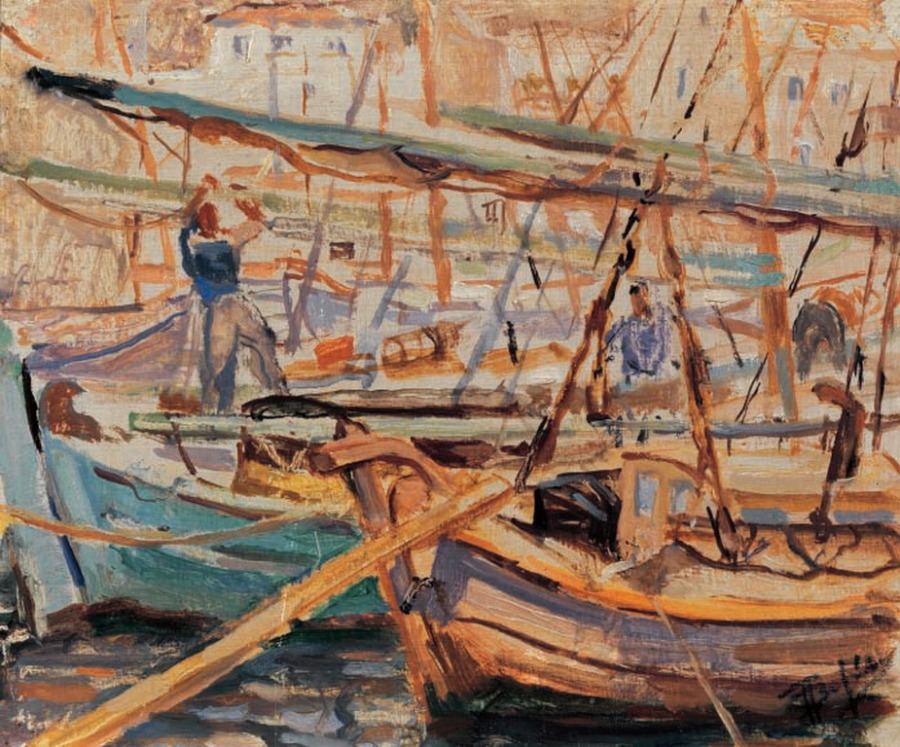This impressionistic painting, evocative of Monet's style, features a dynamic boat dock scene with vibrant colors and abstract forms. In the foreground, a beaten-up, brown and beige wooden boat with blue streaks around the hull, possibly suggesting shadows, is prominently displayed. Tied to the dock beside it is a greenish-teal boat. Both boats have their sails closed. Behind these boats, two men are discernible; the man on the left, dressed in a blue top with red hair, is facing away and appears to be reaching upwards, possibly fixing something. The man in the middle, wearing purple, faces forward, though his facial features are indistinct. Adding life to the scene, a brown dog-like shape is loosely painted nearby. The background bursts with an array of brown, purple, and white shades, alongside abstract representations of sails and houses on a hill, all contributing to the painting's textured composition. The water beneath the boats is a blend of dark black, blue, and tan hues, enhancing the rich complexity of this watercolor-styled artwork.